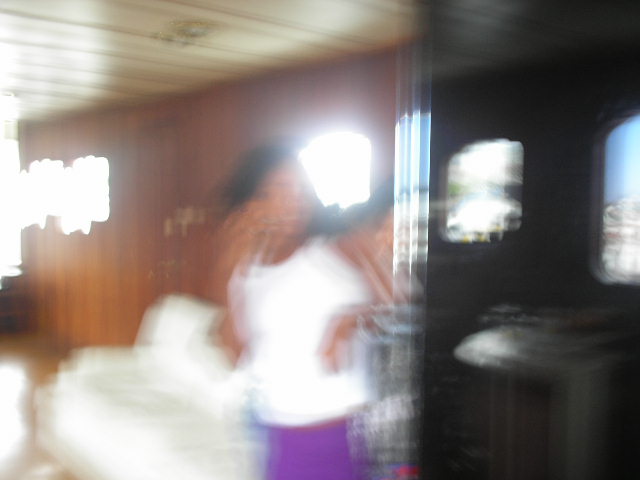In this extremely blurry indoor photo, an indistinguishable woman stands between two rooms. The woman, who appears to be either Black or Hispanic, has black hair. She's wearing a white top paired with eye-catching bright purple pants. The room on the left side of the image features wooden paneled walls and a wooden ceiling, suggesting a rustic or vintage aesthetic. In contrast, the room on the right side has either black walls or walls shrouded in deep shadows, creating a stark dichotomy between the two spaces. Multiple windows are visible in the background, with intense, blinding sunlight streaming through, adding to the motion blur and obscuring any clear details.